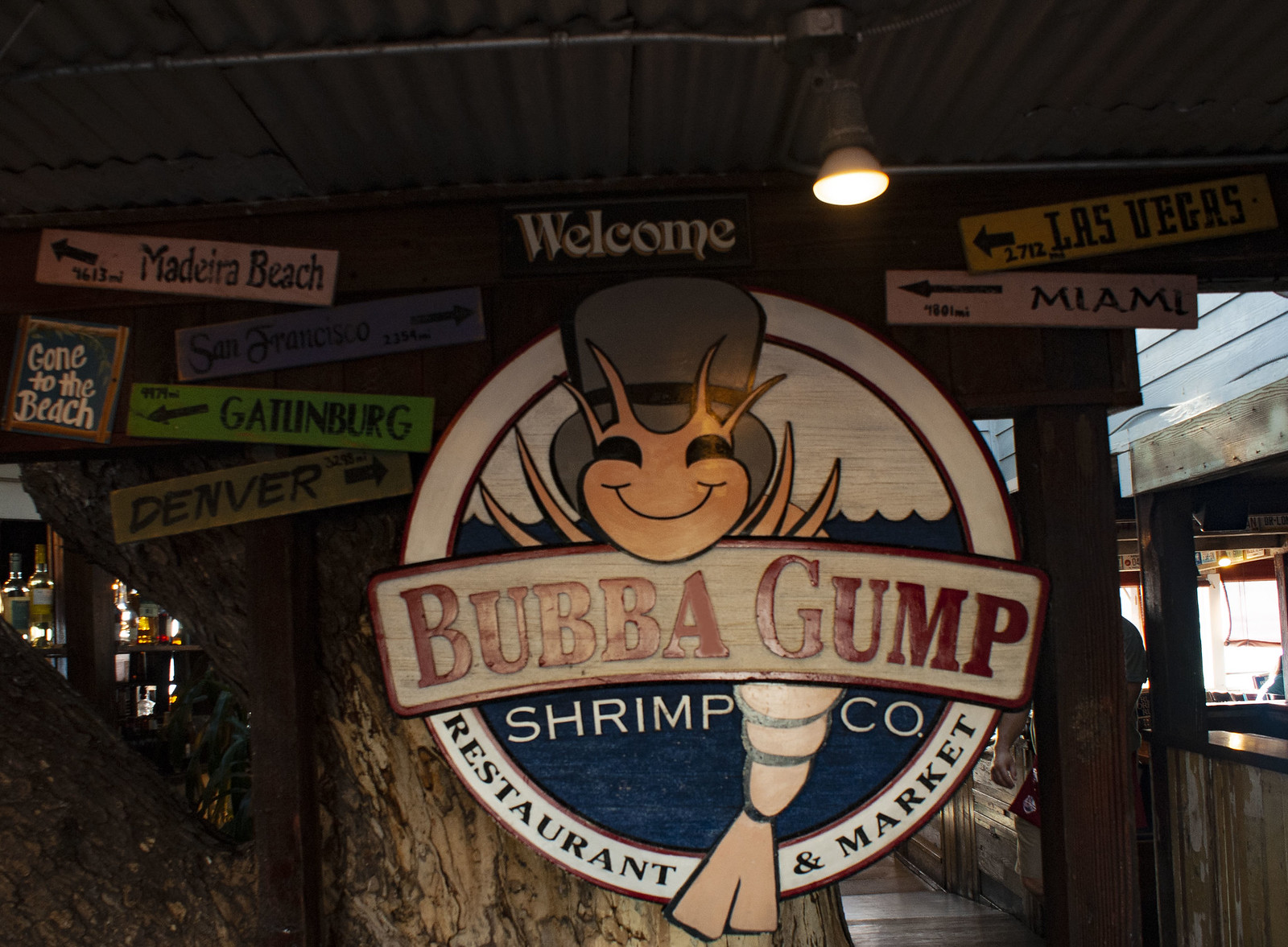The image depicts the entrance signage of the Bubba Gump Shrimp Company restaurant and market. The central element is a large, white circular sign featuring a smiling shrimp wearing a hat, seemingly emerging from blue water, reminiscent of an ocean or lake. Prominently displayed in bold, red letters across the middle of the circle is the name "Bubba Gump," with "Shrimp Co." written just below. The bottom portion of the sign reads "Restaurant and Market." This sign is attached to a wooden background, and above it, there are several directional signs resembling road signs. These include "Welcome," "Madeira Beach," "Gatlinburg," "Denver," "Las Vegas," "Miami," and one additional sign that reads "Gone to the beach." The signage area appears to be under a ceiling made of dark gray metal grates, with a small gray wire and a single light bulb positioned slightly to the right of the center. The overall theme and design elements suggest a playful, nautical atmosphere inviting guests to the establishment.